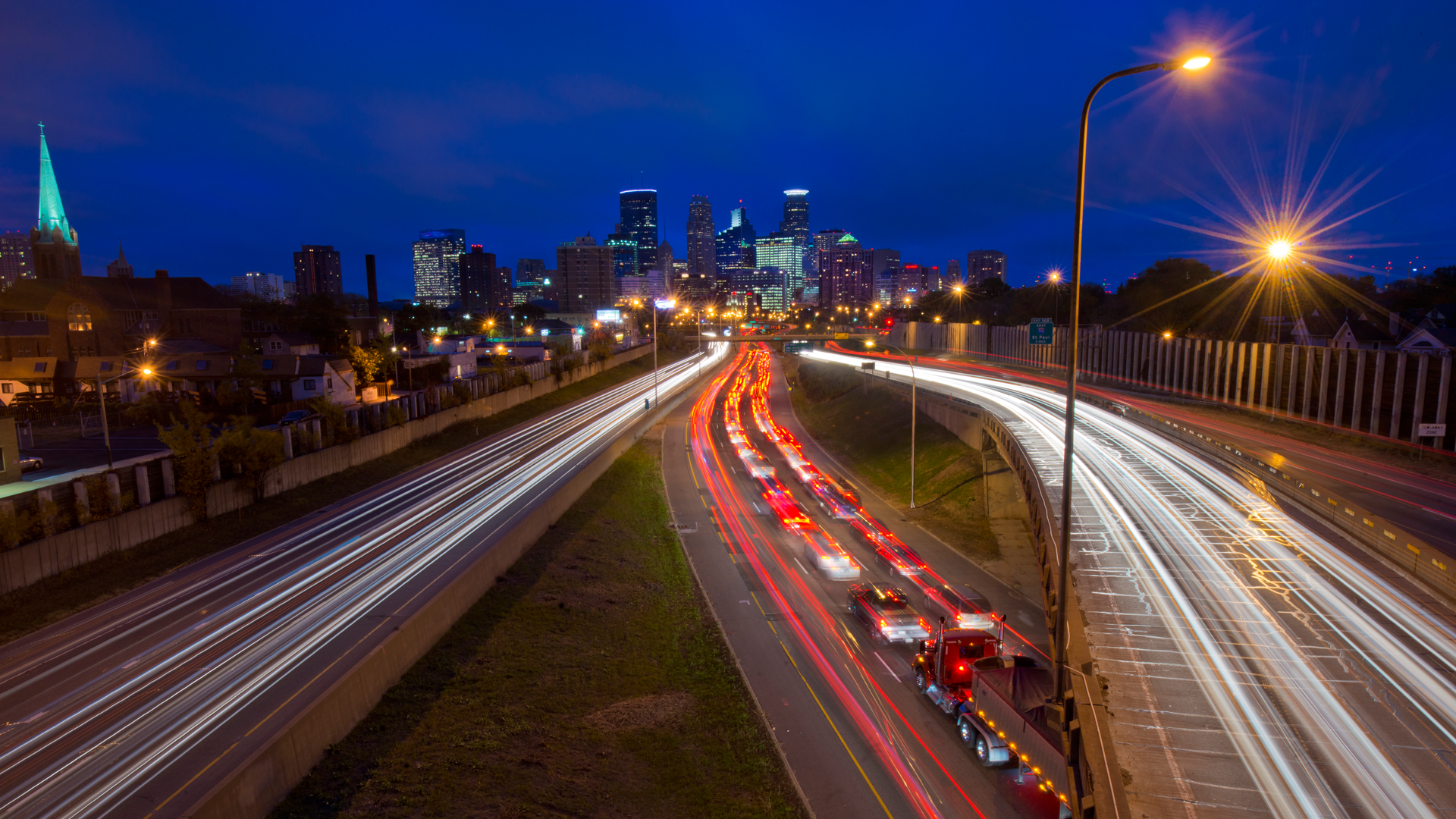The nighttime photograph captures the dynamic motion of traffic on a bustling highway, depicted through the blur of red and white light trails created by vehicle taillights and headlights. Multiple roads intersect and diverge in the scene, including an interstate with an on-ramp and exit ramp. To the right, a bridge arches over the highway, underscoring the intricate design of the urban roadway. In the foreground, a semi-truck is visible among the fast-moving cars. The scene is illuminated by bright streetlights, one positioned beside the bridge and another near the road on the right side. A patch of grass with a small hill can be seen between the roads. In the background, a towering city skyline punctuates the night sky, with buildings adorned in cyan and yellow lights. On the left, the distinctive cyan-colored rooftop of a building stands out. The sky itself is a deep, vivid blue, enhancing the contrasting lights of the city and traffic.